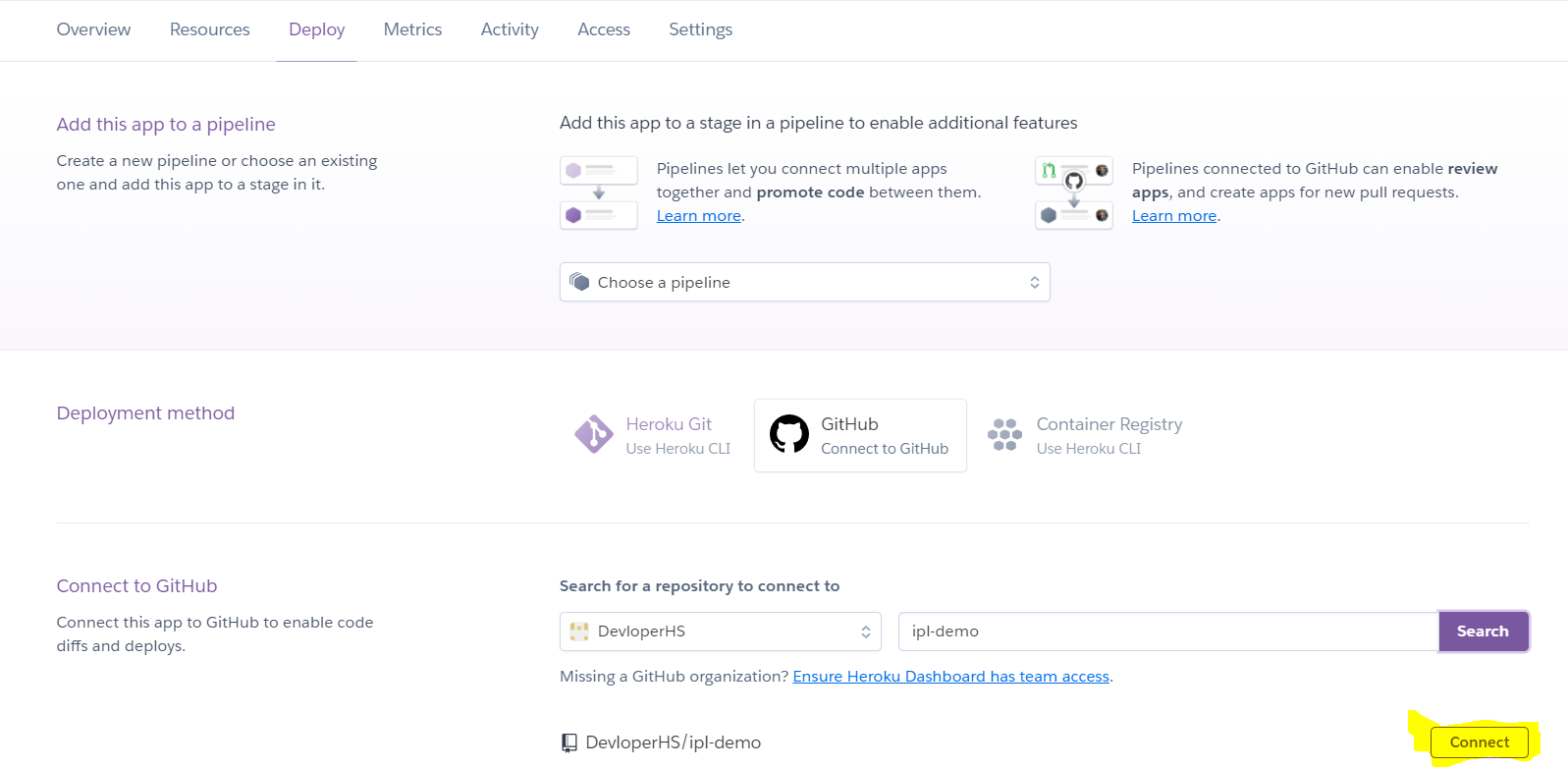The interface displayed offers a suite of options housed in multiple buttons at the top, labeled as Overview, Resource Deploy, Matrix, Activity, Access, and Settings. Currently, the interface is focused on the 'Deploy' section, highlighted by an underline. 

Below this navigation bar, on the left, there's an instruction to "Add this app to a pipeline." Users are prompted to either create a new pipeline or choose an existing one for addition to the stage. 

Adjacent to this, on the right, further instructions suggest adding the app to a stage in a pipeline to enable different features. This section illustrates the process with a series of icons and arrows, visually guiding the user through the sequential steps. It emphasizes that pipelines connect multiple apps enabling code promotion between them. An option to learn more is also provided.

Below these instructions, users are invited to "choose a pipeline," displayed via a drop-down menu that offers various pipeline options. Beneath this, the deployment method section presents Heroku Git, Kit, and GitHub options. 

Particularly, for GitHub users, there's an option to "Connect to GitHub," facilitating code drifts and deployment. A search repository feature is available, currently set to "developer HS," but this can be changed. A search bar is located nearby, and at the bottom right, a prominent yellow button labeled "Connect" stands out.

The background of the interface is predominantly white, with the text mostly in black, ensuring clear readability.